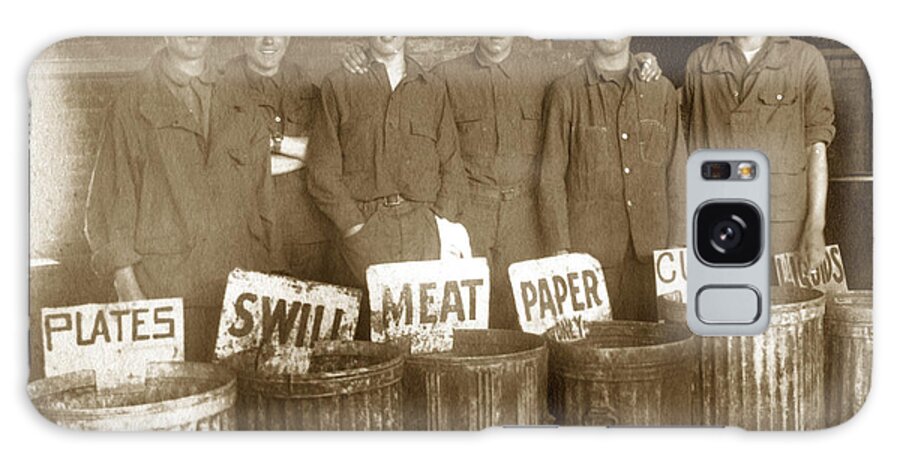This image, used as a phone case, showcases a vintage black-and-white photograph depicting six men in dark, perhaps grey, jumpsuits or uniforms. The men are visible only from the nose downward, and they appear to be white, all standing in a row behind old, silver trash cans. Each can is labeled with a white paper indicating "plates," "swill," "meat," "paper only," and "liquids," while one label is obscured. The image is horizontally positioned on the phone case, with the phone’s camera lens and flash prominently visible in the middle of the composition. The background reveals some walls, adding to the vintage feel of the photograph.